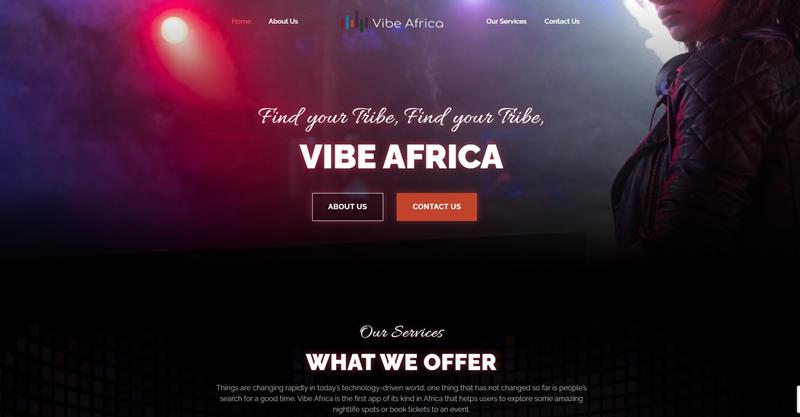This image depicts a dark-themed screenshot from an application with a red light illuminated near the top-left corner. The partial view of a woman is visible, with her looking over her left shoulder, though the top part of her face is not shown. The text at the top of the screenshot includes navigation headers reading, "Home," "About Us," "Vibe Africa," "Our Services," "Contact Us," "Find Your Tribe," repeated twice, "What We Offer," among others. An informational paragraph describes Vibe Africa as a pioneering app on the continent, enabling users to discover nightlife experiences and book event tickets, emphasizing the human desire for enjoyment even amid rapid technological change. The screenshot is devoid of any animals, buildings, birds, plants, vehicles, or natural landscapes like mountains.